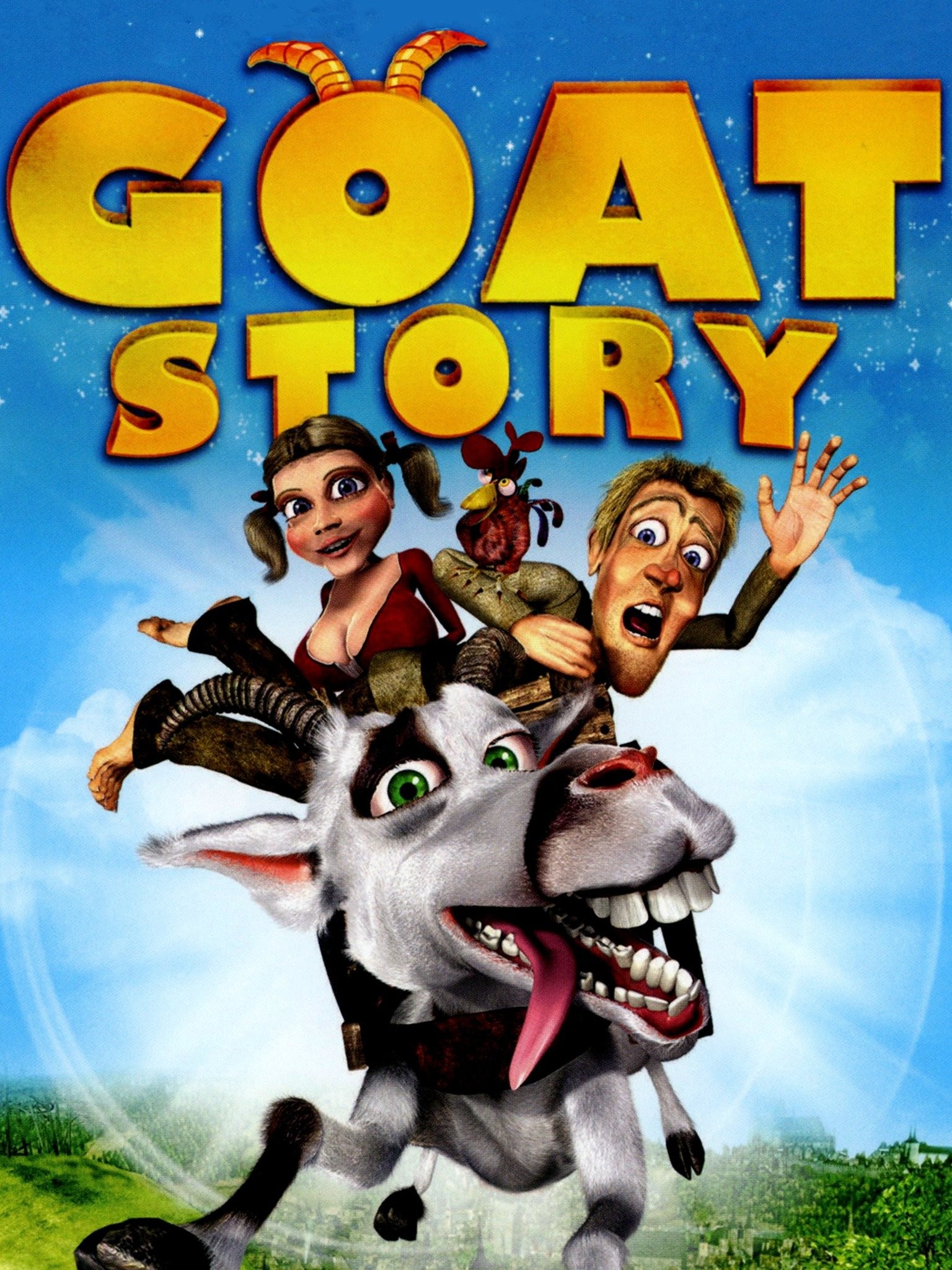The image appears to be a vertical rectangular poster, likely for a movie titled "Goat Story," derived from the large yellow text at the top displaying the word "GOAT" with distinctive horns protruding from the letter 'O.' Below the title, in slightly smaller yellow letters, is the word "Story." The poster features a whimsical, animated scene. Central to the image is a large white goat with green eyes and striking, dark brown horns; its mouth is agape, revealing prominent teeth with its tongue lolling to the left.

Riding on the goat's back are two animated characters. To the left is a cartoonish woman with brown hair styled in pigtails, wearing a red shirt. She sits behind the goat’s head, her expression wide-eyed and exaggerated. Next to her, slightly sprawled across her lap, is a man with a comically surprised expression, his right hand up as if trying to grasp something, while a small bird perches on his right arm.

The scene is vibrant, with a backdrop of a blue sky and a splash of sunlight. Green grass and bushes frame the bottom of the image, and the goat appears to be in motion, contributing to the chaotic and humorous atmosphere. The overall impression is one of dynamic action and playful absurdity, capturing the lighthearted essence of the story being advertised.